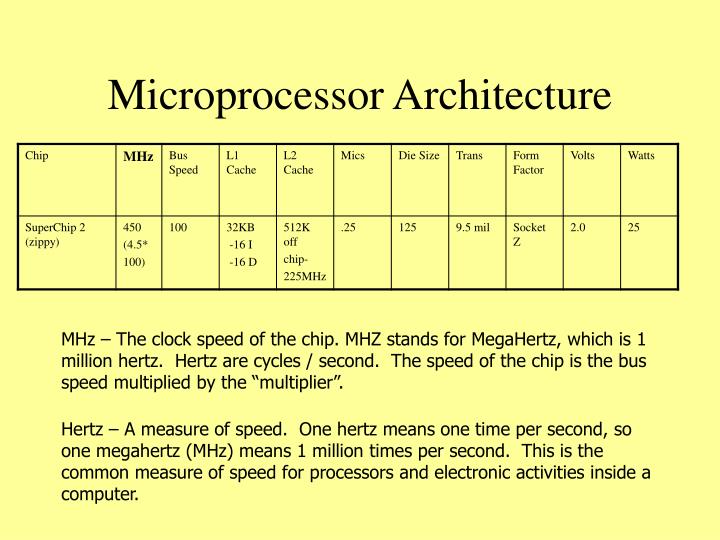In the image, a light yellow rectangular box prominently displays a detailed informational chart titled "Microprocessor Architecture" in bold black text at the top. The chart, divided into two rows and approximately twelve columns, includes information about various technical specifications such as chip details, bus speed, and cache. Below the chart, black text explains technical terms: MHZ (megahertz), the clock speed of the chip, defined as one million hertz or cycles per second. Additional definitions are partially visible. The overall layout and structured content suggest that the image could be part of a larger poster or informational slide, likely used in educational or professional presentations.